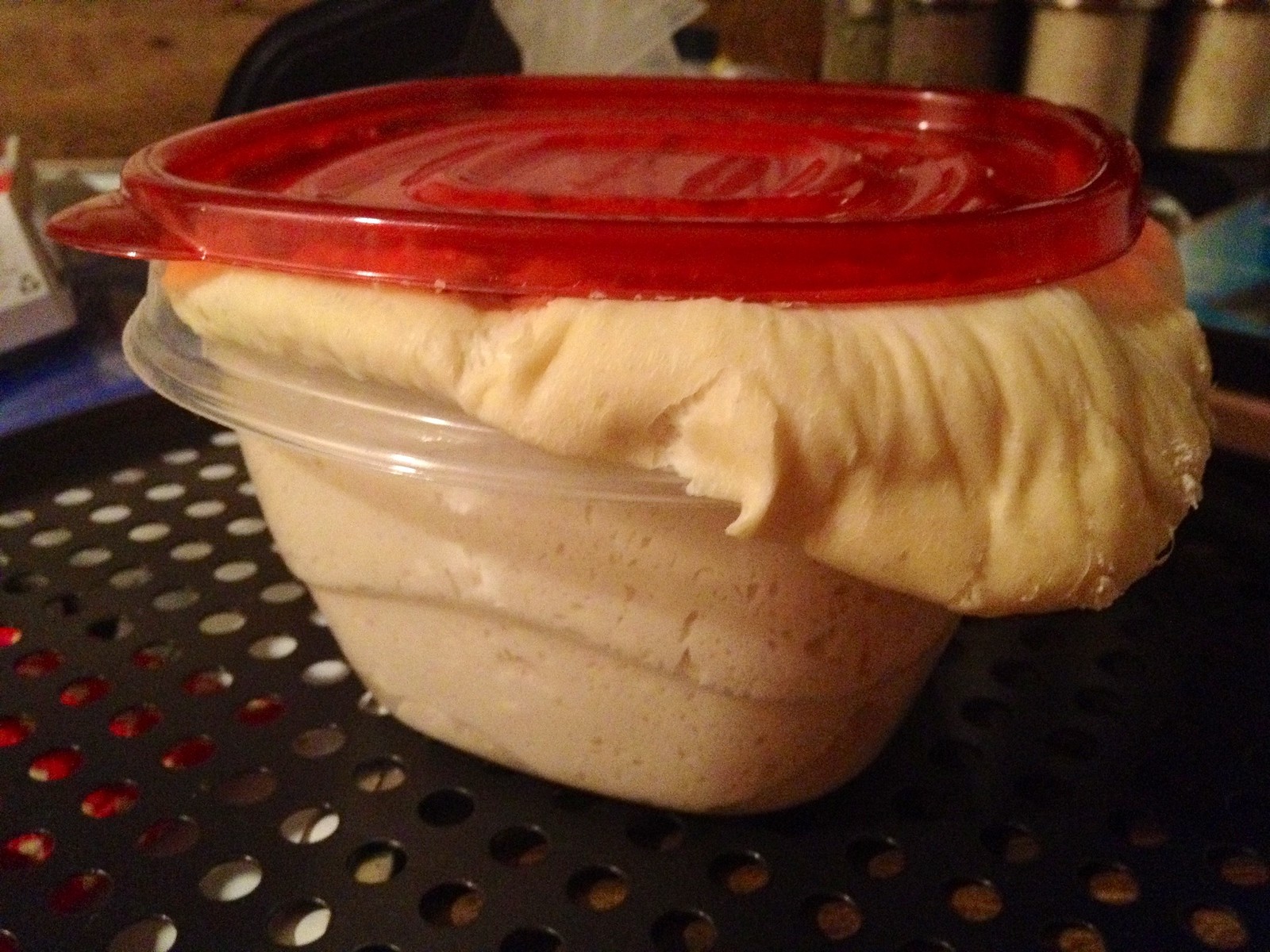In this image, a clear, square-shaped Tupperware container with a red lid is visibly overflowing with a light, dough-like substance that has risen beyond the container’s capacity. The contents spill slowly over the sides, hinting at a yeast-like expansion. The container sits on a black, perforated tray that resembles a grate or drainage device, covered in small, evenly spaced holes. The tray is situated in the foreground, while the background displays a wooden wall and a black office chair. To the left of the scene, a purple surface holds a box, adding a subtle color contrast to the setting. Notably, the lid of the container appears to have a small amount of dust in its center. The dough inside is pale, reminiscent of vanilla or lightly colored pastry, offering a stark contrast to the dark tray beneath.